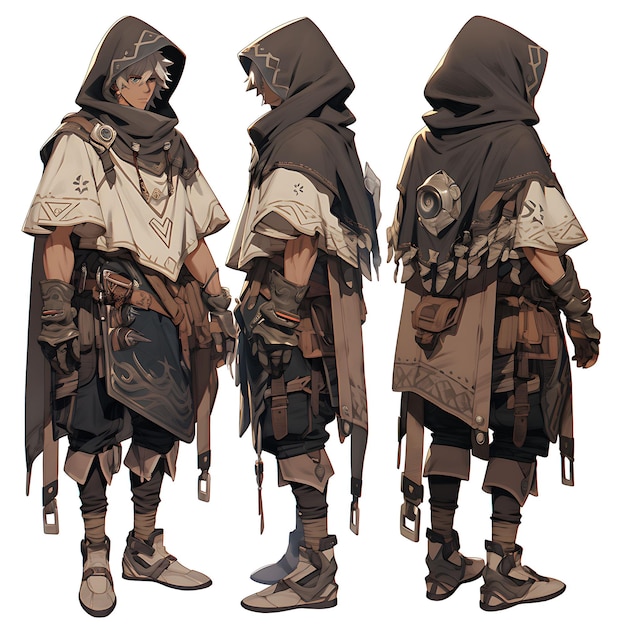This image features a detailed character design of an anime figure displayed from multiple angles: front, side, and back views. The character is dressed in a cream-colored cloak adorned with triangle symbols, and sports a brown headdress that allows visibility of their sharp-featured face, with spiky blonde hair. Their arms appear muscular, clad in brown leather gloves. 

The side view reveals more specific details, including capri-style black pants with visible straps, brown socks, and brown boots accented with darker shades. The back view uncovers additional elements like a round metal piece on the cloak and straps with metal buckles hanging down. Despite appearing to be different characters, each angle actually represents the same character silhouetted against a blank white background. Noticeably, this character embodies a blend of strength and mystery, reminiscent of a cloak-and-dagger aesthetic, with an attire suggestive of secretive or adventurous roles marked by practical and distinctive accessories such as the sheathed side knives and a hooded cape.